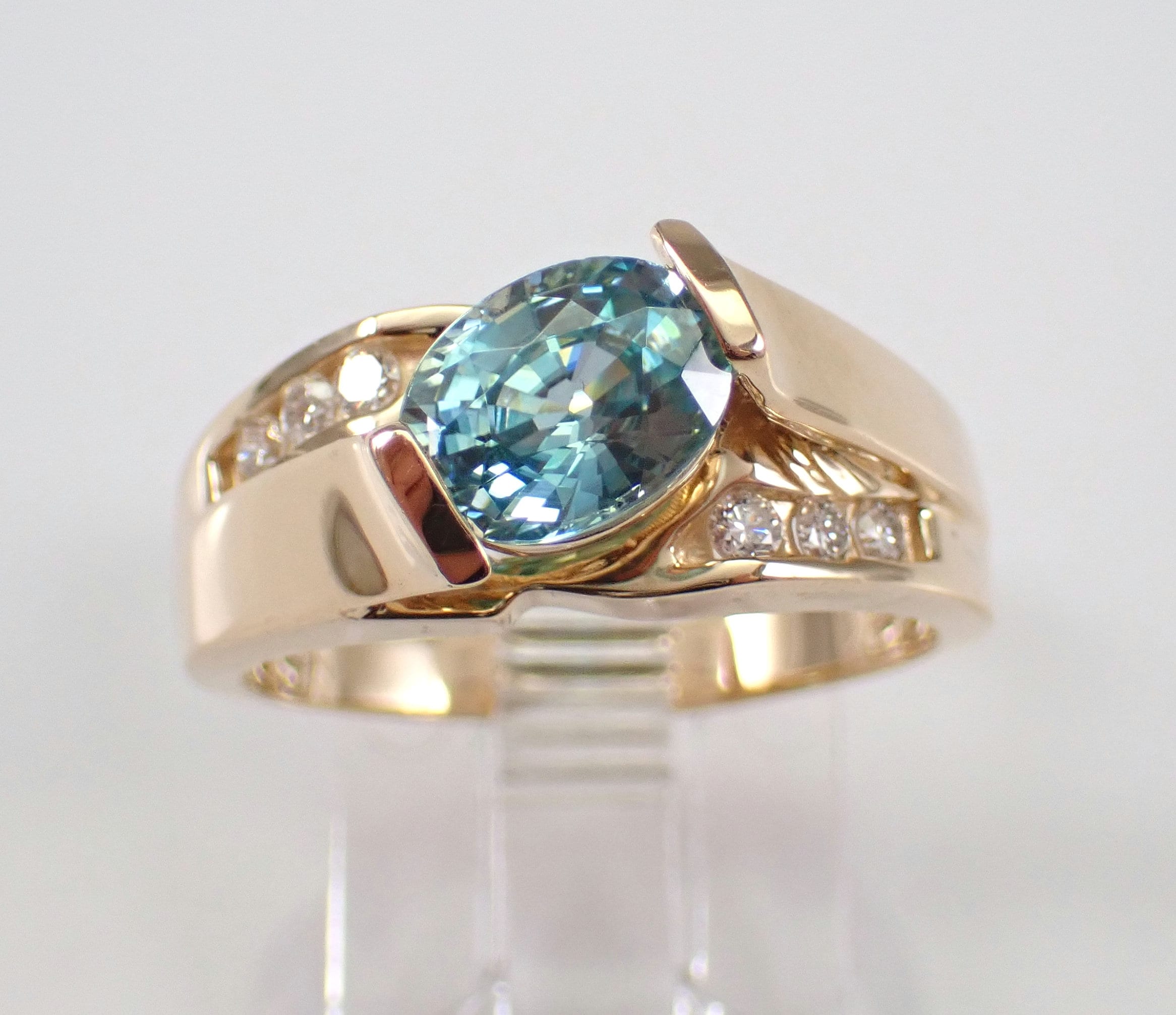This professional photo features a striking gold diamond ring displayed on a transparent plastic stand. The centerpiece of the ring is an eye-catching, light blue diamond with an oval cut, brilliantly reflecting light from multiple angles. The gold band is designed to elegantly cradle the blue diamond, coming up on either side to secure it. Intricately placed on both the right and left sides of the central gemstone are clusters of three smaller white diamonds, adding to the ring's allure. Notably, there is a brown strip on the left side of the band, near where it supports the main diamond. The entire scene is set against a pristine, white background, ensuring that every detail of the ring's craftsmanship is vividly displayed.